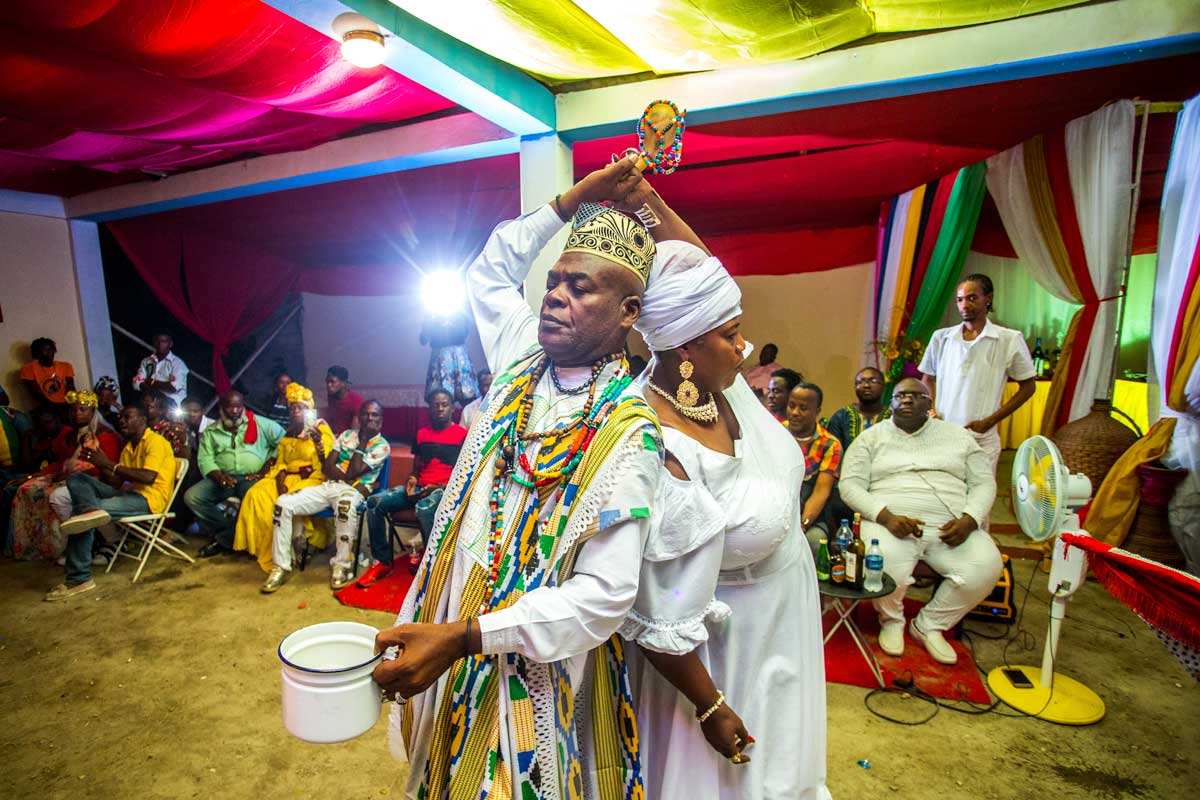In this vibrant color photograph, an African man and woman are captured in the midst of a ceremonial dance within an indoor venue designed to evoke the interior of a tent. Both are adorned in traditional white robes, with the man wearing an ornate hat of gold and black, and the woman donning a white head wrap and a striking earring featuring two gold circles, the larger one accented by a dark dot. She also wears a golden necklace and has her right hand adorned with red fingernail polish. They stand back-to-back, their clasped hands raised above their heads, holding a beaded emblem, while the man’s left hand holds an open white bucket with a black rim. Surrounding them are over 20 spectators of African descent, some watching intently, others partially engaged with different activities. The room, with its white walls, fabric ceiling, and drawn-back curtains, is decorated with silky scarves and fabric. A standing oscillating fan with a white exterior and yellow blades is visible on the right side, indicative of the warm environment. The scene captures the attention of the crowd, many of whom have their phones out, documenting this cultural celebration.